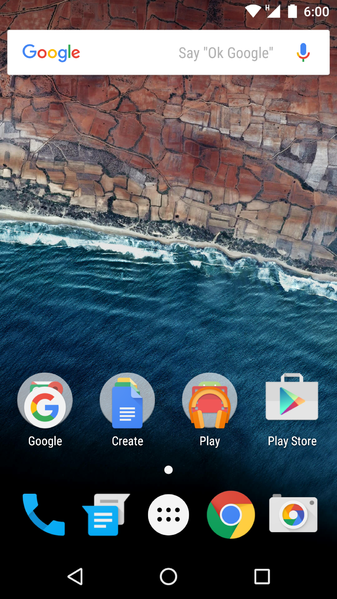This image is a screenshot taken from a smartphone. The upper right corner of the screen displays the time in white font, which reads 6:00. The battery icon indicates that the phone is fully charged. The background image is beautifully split between the upper half of the screen, showcasing rugged cliffs with textured rocks in dusty pink, gray, and steel gray hues, and the bottom half featuring mesmerizing deep blue water.

At the bottom, there are two rows of app icons. On the first row, from left to right, we see:

1. The Google app icon represented by the letter "G."
2. A blue schematic drawing of a piece of paper labeled "Create."
3. An app labeled "Play," with an icon that resembles an orange cat.
4. The Google Play Store icon, which looks like a multicolored pyramid.

On the second row, from left to right, we see:

1. The phone icon in turquoise blue.
2. The messaging app icon, also in turquoise blue.
3. The Google Chrome logo.
4. The camera app icon.